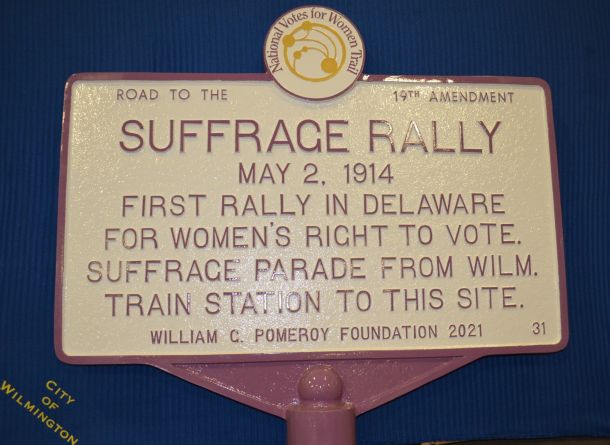This image showcases a signpost against a deep blue background, with "City of Wilmington" inscribed in the lower left-hand corner. The sign, appearing somewhat aged, is supported by an arch in a rose pink color and contains significant historical details. At the top of the sign is a blue circular badge that reads "National Votes for Women Trail," with an inner circle featuring yellow drawings and patterns. The main rectangular section of the sign has a cream-colored background framed by the same rose pink hue. The text, also in rose pink, reads: "Road to the 19th Amendment, Suffrage Rally, May 2nd, 1914. First Rally in Delaware for Women's Right to Vote. Suffrage Parade from Wilm. train station to this site. William C. Pomeroy Foundation, 2021." The number "31" is displayed in the lower right-hand corner of the sign. Overall, the sign commemorates a historic women's suffrage event held in Wilmington.